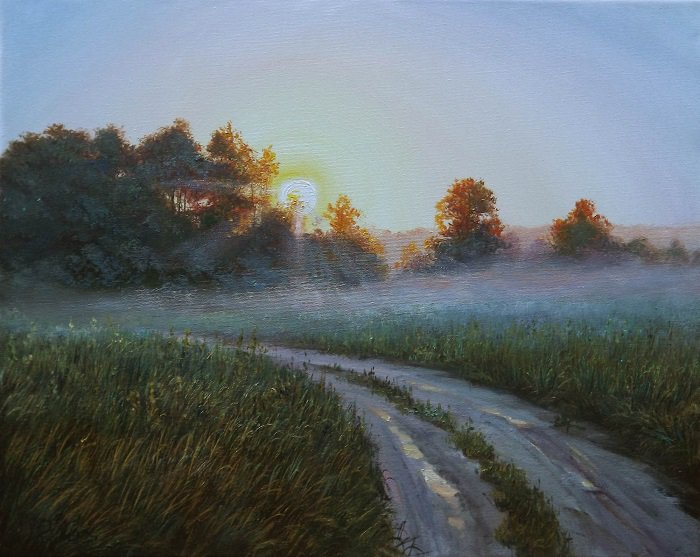A serene and tranquil early morning scene unfolds in this picture, featuring a country road framed by lush greenery. Tall grass lines the path, bisected by tire tracks that form a rustic road leading into the distance. The soft, golden light of the rising sun filters through the trees in the background, casting a gentle haze over the landscape and enhancing the peaceful atmosphere. The sky above is clear and blue, completing the idyllic setting.